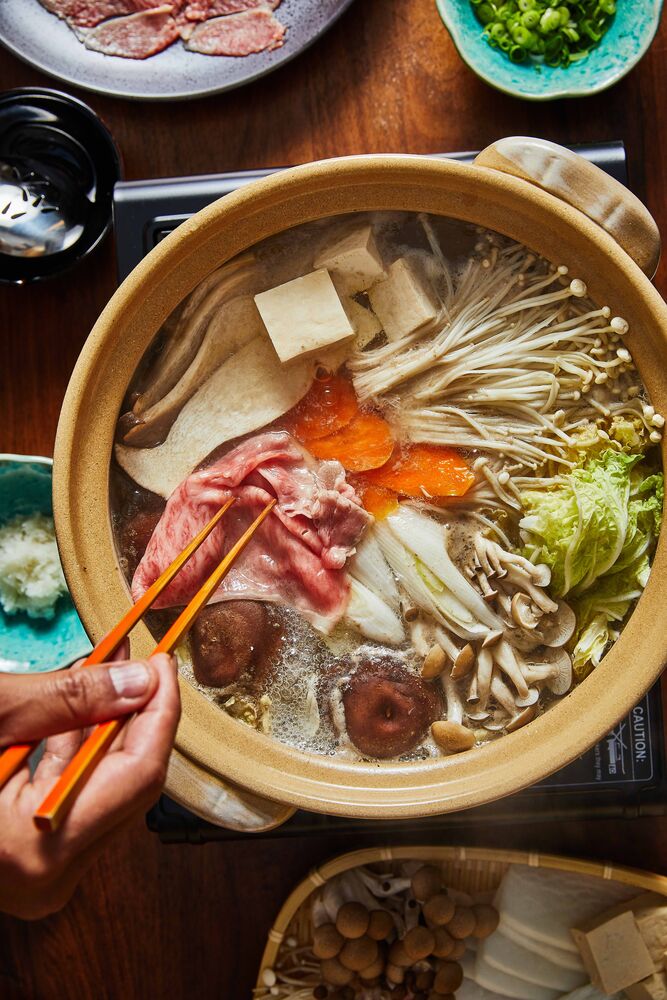A top-down shot captures a vibrant, Japanese-style hot pot in a tan-colored bowl, adorned with an array of ingredients. The steaming broth is filled with cubed tofu, three different kinds of mushrooms, enoki among them, sliced carrots, cabbage, and thinly sliced wagyu beef. A hand with a light brown skin tone enters from the bottom left, poised with orangey-brown wooden chopsticks, ready to grasp the tender beef. The bowl rests on a dark brown wooden table cluttered with additional food items and condiments. Adjacent to the hot pot, a plate brimming with similar ingredients waits to be added, and a big serving spoon lies nearby, amidst the culinary assortment. The surrounding scene includes glimpses of other plates and containers, enhancing the banquet's warm, communal atmosphere.